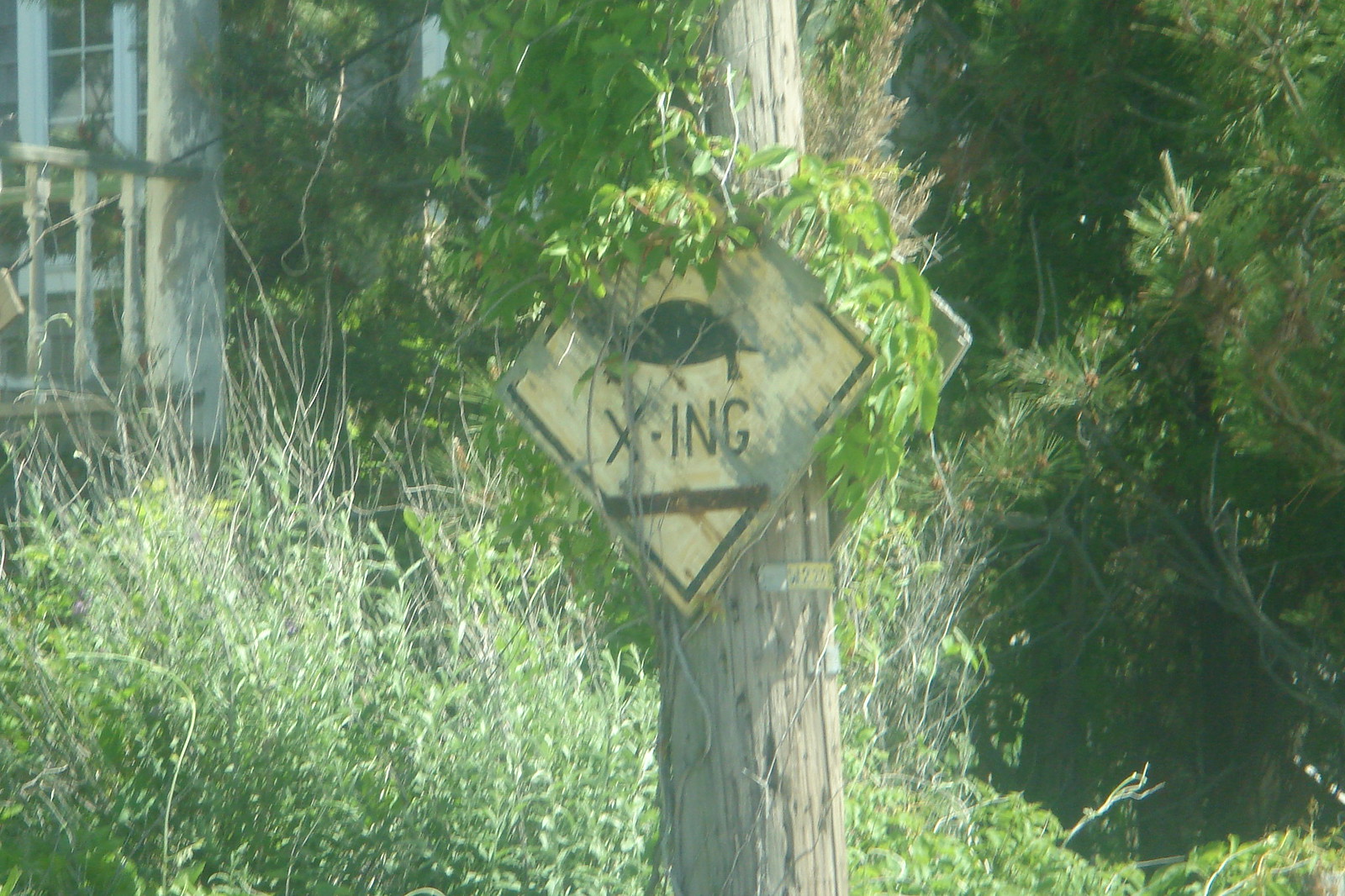This image captures a somewhat neglected backyard and adjacent wooded area. On the left side, there's an older house featuring a porch and white-window frames. The lawn is heavily overrun with weeds, grasses, and various brushes. In the central part of the image stands an aging telephone pole adorned with a distinctive yellow diamond-shaped sign, which bears the silhouette of a black turtle and the text "XING," indicating a turtle crossing. The sign appears faded and is partially covered by vines. To the right, the scene transitions into dense foliage with pine trees and overgrown vegetation. Additionally, the telephone pole has a metal tag with numbers that are difficult to discern. The overall scene suggests an area where turtles may be native and frequently cross, with a need to alert passersby to their presence.